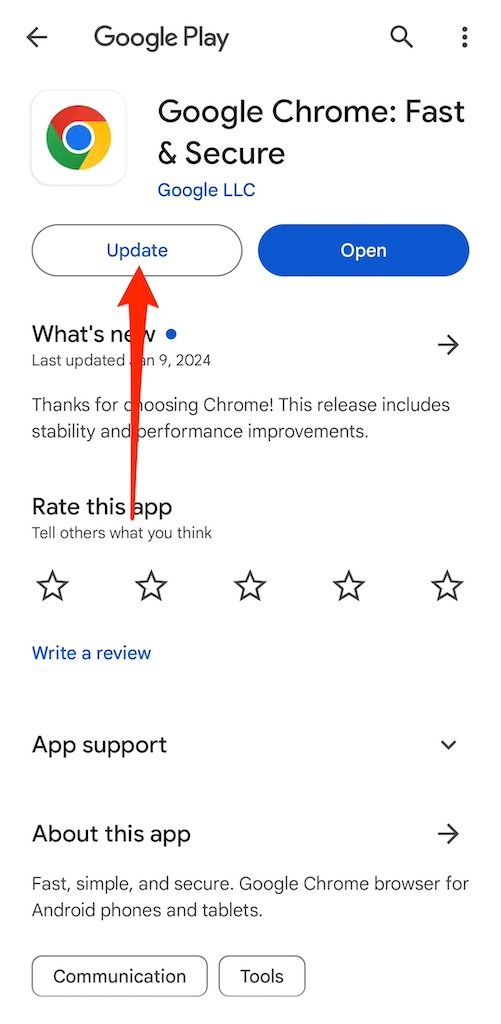This image depicts the Google Chrome browser app page on the Google Play Store as viewed on a mobile device, such as a phone, tablet, or Chromebook. At the top of the screen, the header reads "Google Play," indicating the app store's platform.

Below the header is the listing for the Google Chrome browser, officially titled "Google Chrome: Fast & Secure" and developed by Google LLC. Centered beneath the app title and developer name, two buttons are prominently displayed. An arrow, added through a paint program, points to the button on the left labeled "Update," suggesting that the user has the app already installed and needs only to update it. The button to the right, labeled "Open," allows the user to directly launch the Google Chrome app from this screen.

Further down, there's a section for rating the app, which the user has not yet utilized, indicated by the absence of any submitted ratings. The "What's New" section notes, "Thanks for choosing Chrome. This release includes stability and performance improvements." Additional options include a dropdown menu for app support and a button linking to the "About" page for more detailed information about the Google Chrome browser.

Finally, at the bottom of the description, the app is categorized under "Communication" and "Tools" on the Google Play Store.